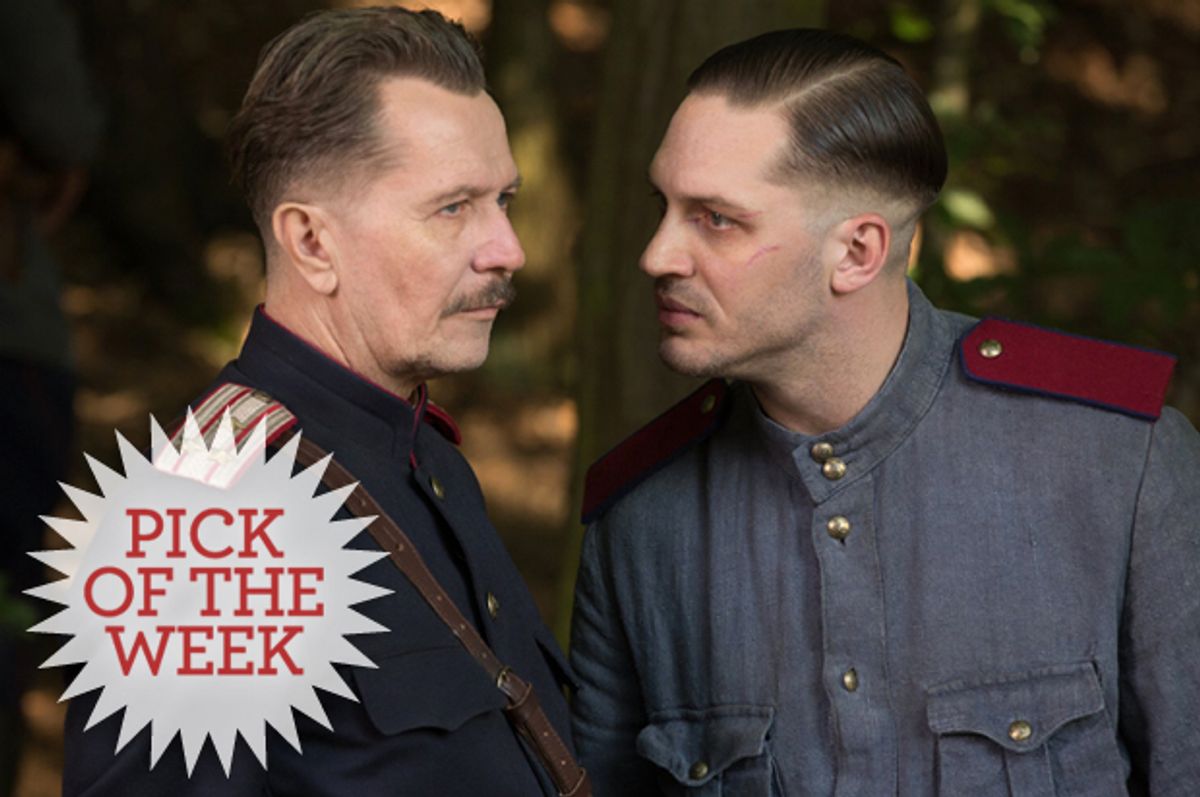This detailed image captures actors Gary Oldman and Tom Hardy in a striking scene, likely from a movie set during the World War II era. The still features both men in historically inspired military uniforms. Gary Oldman, on the left, stands with a calm yet stern demeanor, gazing off into the distance. His light brown hair, styled and slightly receding, frames his weathered, mustached face, accentuated by a prominent forehead and sharp features. He dons a dark blue wool military jacket adorned with brass buttons and white-and-maroon shoulder pads, with a brown leather strap crossing his chest.

Tom Hardy, positioned to the right, contrasts with a more intense and focused expression, his glare seemingly directed at Oldman. He sports a clean-shaven look, his light brown hair slicked down, and his face marked by a few small scratches. Hardy's uniform is a bluish-gray color with maroon shoulder straps and matching brass buttons. 

Enhancing the focal point of the composition is a spiky white starburst in the foreground, emblazoned with "Pick of the Week" in bold red lettering. This stylistic element overlays the image, paired with a similar watermark at the bottom left, reinforcing the importance of this memorable cinematic moment.